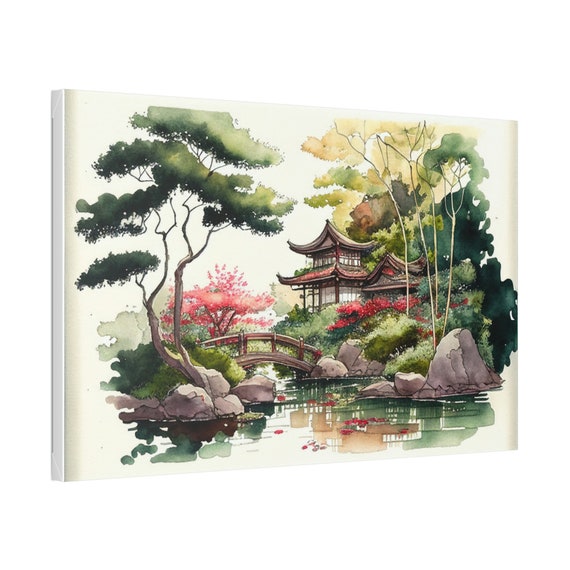The image features a detailed water-painted depiction of a serene Japanese garden from feudal Japan. Dominating the background is traditional Japanese architecture, showcasing distinctive curved roofs and clear panels, indicative of an old-style house surrounded by an abundance of greenery. A picturesque walking bridge connects this structure to another island, enhancing the scenic charm with its graceful span over clear, green water streaked with shades of red, reflecting rose petals nearby.

Cherry blossoms and bonsai trees add undeniable beauty and tranquility, scattered throughout the canvas, their blossoms appearing both in the trees and the water below. Gray rocks dot the landscape, contributing to the natural, rugged contrast against the lush vegetation. On one side, the trees are vividly painted in shades varying from deep green to a lighter hue, while distant, impressionistically blotched trees add depth and texture. The peaceful ambiance, reminiscent of scenes from "Memoirs of a Geisha," accentuates the garden's harmonious blend of nature and traditional architecture.